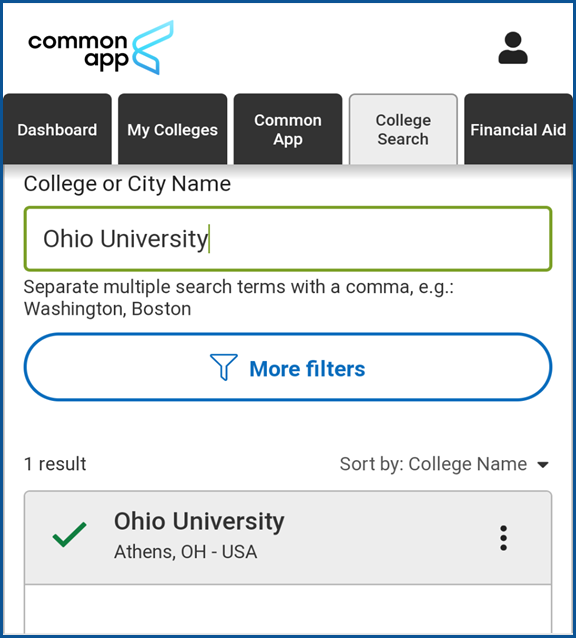### Descriptive Caption for the Common App Screenshot:

The screenshot displays the user interface of the Common App, a platform primarily used for submitting college applications. At the top left corner, a light blue, wavy symbol represents the Common App logo. Adjacent to the logo is a nondescript icon. Below the header are various navigational tabs: "Dashboard," "My Colleges," "Common App," "College Search," and "Financial Aid." These tabs are black with white text, except for the "College Search" tab, which is currently active, making it white with black text.

Upon selecting "College Search," the interface displays a search bar at the top, where "Ohio University" has been entered. This search bar is outlined in green, with the cursor also appearing green inside it. Beneath the search bar is an instructional note: "Separate Multiple Search Terms with a Comma," accompanied by an example using "Washington, Boston."

A blue button labeled "More Filters" is available below the search bar for additional search options. The search results indicate one result for "Ohio University," marked by a green checkmark. Additional details include its location: Athens, Ohio, U.S. To the right of this result, there are three dots, offering more information about Ohio University.